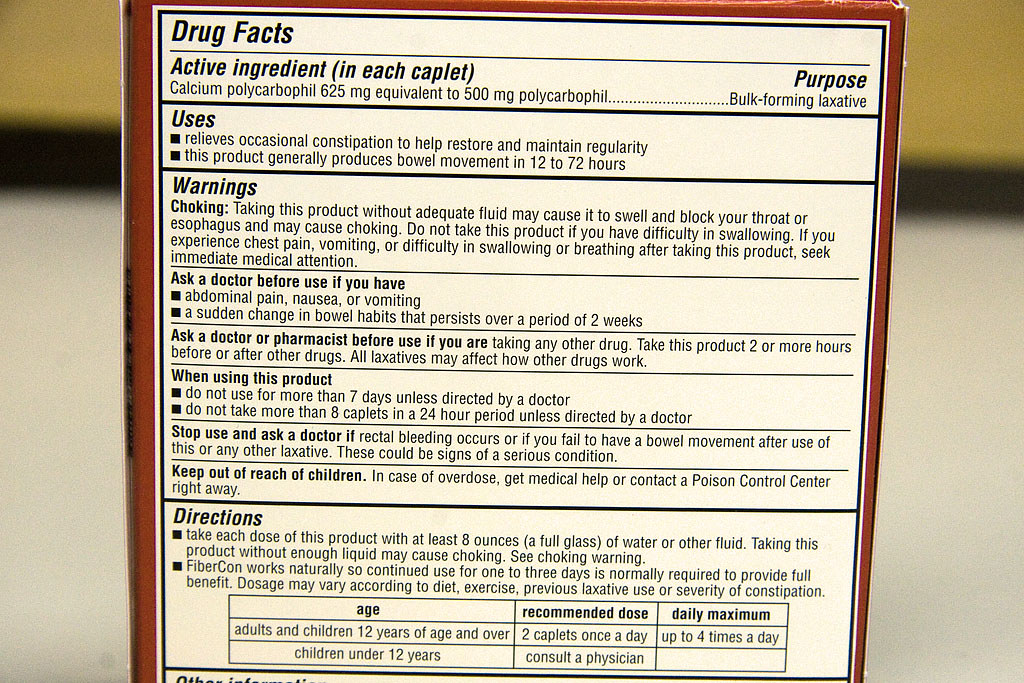This image displays the "Drug Facts" section on the back of a brownish-red outlined medicine box, predominantly featuring a white background. The top of the image has a blurred yellow section with a black line, while the bottom three-quarters is covered in white. The main focus falls on a detailed white panel which lists various information in black text.

At the top of the panel, the label "Drug Facts" is prominently displayed, followed by details on active ingredients, specifically noting that each cathlet (tablet) contains 625 milligrams of calcium polysaccharide, equivalent to 500 milligrams of polycarbophil, a bulk-forming laxative. 

Under the active ingredients, the "Uses" section mentions that the product is intended to relieve constipation, typically producing a bowel movement within 12 to 72 hours. 

A warning section follows, cautioning users about the risk of choking and advising them to consult a doctor if experiencing symptoms such as abdominal pain, nausea, vomiting, or sudden changes in bowel habits that persist over two weeks. Additionally, it warns against using the product for more than seven days or taking more than eight cathlets in a 24-hour period, and to stop use if no bowel movement occurs after use. 

The directions indicate that children aged 12 and over should take two cathlets once a day, with a maximum of four doses per day, while children under 12 should consult a physician. It also highlights the importance of consuming the cathlets with eight ounces of water.

The bottom of the panel includes a reminder to keep the product away from children, alongside numerous other details that are not fully visible in this image.